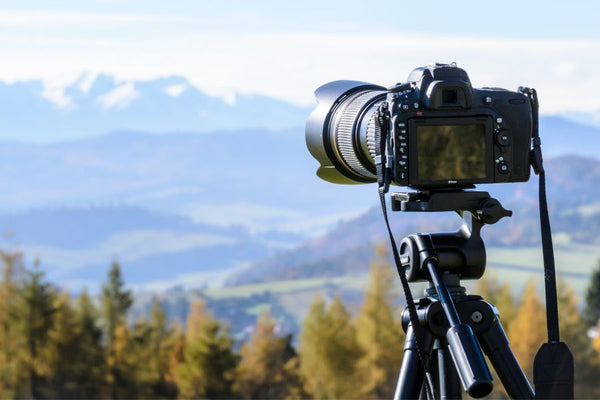In this detailed image, a black professional camera is set up on a tripod, aiming at a stunning mountain scene. The camera, equipped with a large lens and straps hanging from either side, captures a picturesque landscape. The viewpoint is from behind the camera, where you can see its screen and various buttons. The scene includes a lush green valley surrounded by dense forestry of pine trees. In the distance, the majestic snow-covered peaks of a mountain range rise under a beautiful blue sky dotted with clouds. The camera's position right at the edge of a cliff offers an expansive view of the countryside, making it evident that the photographer has carefully chosen this vantage point to capture the breathtaking scenery. All components, from the vibrant meadows in the valley to the towering white mountains, contribute to the image's panoramic depth and natural beauty.